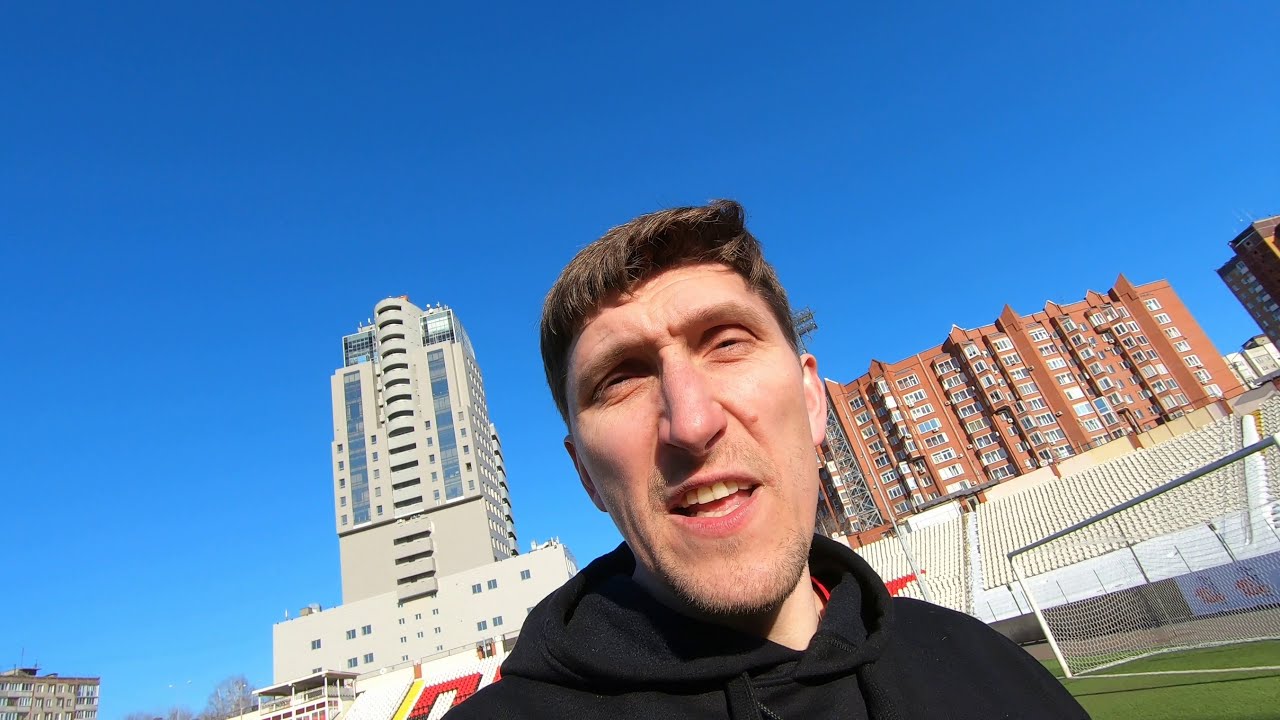In this image, a man is taking a selfie on what appears to be a soccer field, likely on a college campus. The man, who is Caucasian with short brown hair and subtle bangs, is squinting into the sun, resulting in an illuminated face. He has a long, narrow face, characterized by a long, straight nose, thin pink lips, and some light-colored stubble on his chin and above his upper lip. He is wearing a black hoodie and is captured with his mouth open, revealing his top teeth, suggesting he is talking. 

The background features a vivid blue sky and several buildings: to his right is a red-brick, multi-story building that might be an apartment or dormitory, and on the left is a taller, tan-gray sandstone skyscraper. Additionally, there's a soccer goal with a net visible on the green astroturf field, accompanied by empty bleachers that appear to display the name of the school, partially obscured with hints of letters like 'D' or 'O'. The overall composition of the photograph is slightly diagonal and imperfect, consistent with the nature of a selfie or a screen grab from a video.